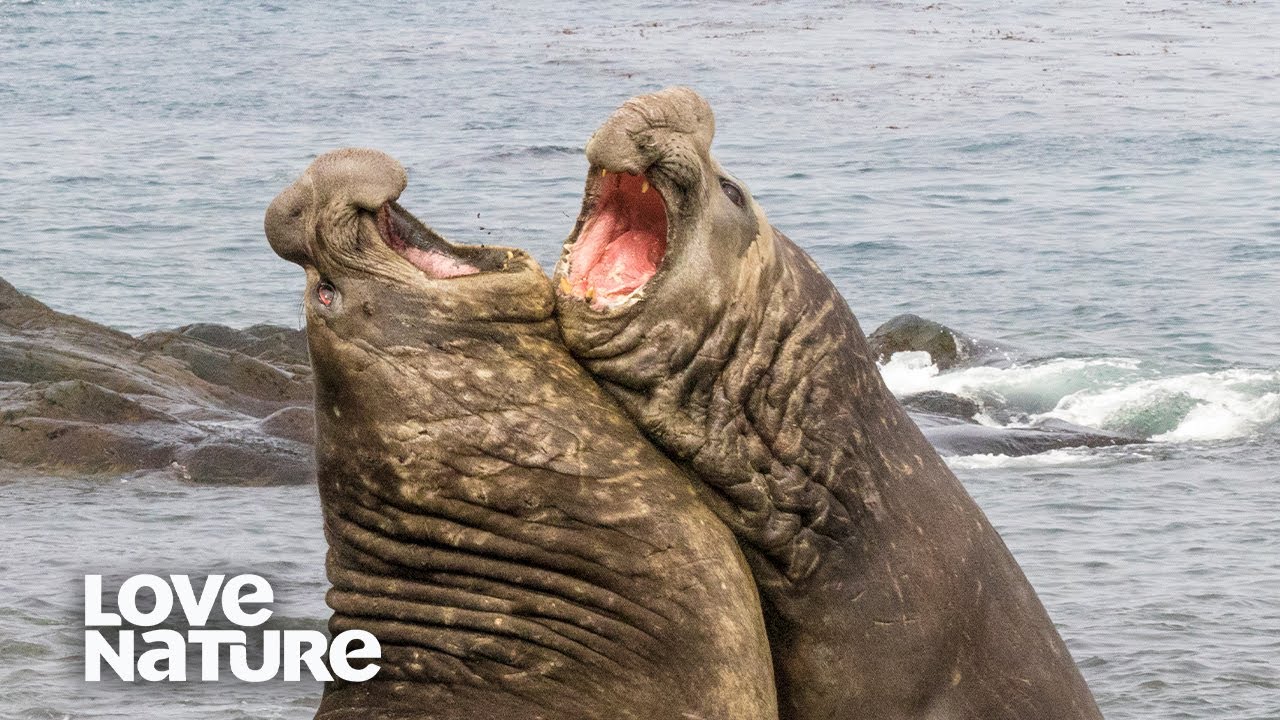The image is a color photograph that appears to be a poster, featuring two large elephant seals. These massive creatures, identifiable by their distinctive large fleshy noses, are seen upright, seemingly embracing or abutting each other. Both elephant seals have their mouths wide open, displaying red mouths with relatively small teeth. The photograph has "Love Nature" written in large, thick white text in the bottom left corner. 

The backdrop consists of an ocean scene with waves and rock outcroppings, giving the impression that the seals are at the seashore, basking in the sunlight. The water and the rocks create a natural, well-lit setting, suggesting the photo was taken in the middle of the day. The overall composition, with the sea creatures set against the seascape, gives a sense of tranquility and the raw beauty of nature. The humorous and seemingly affectionate pose of the seals adds a touch of whimsy to the image, aligning with the message to appreciate and love nature.